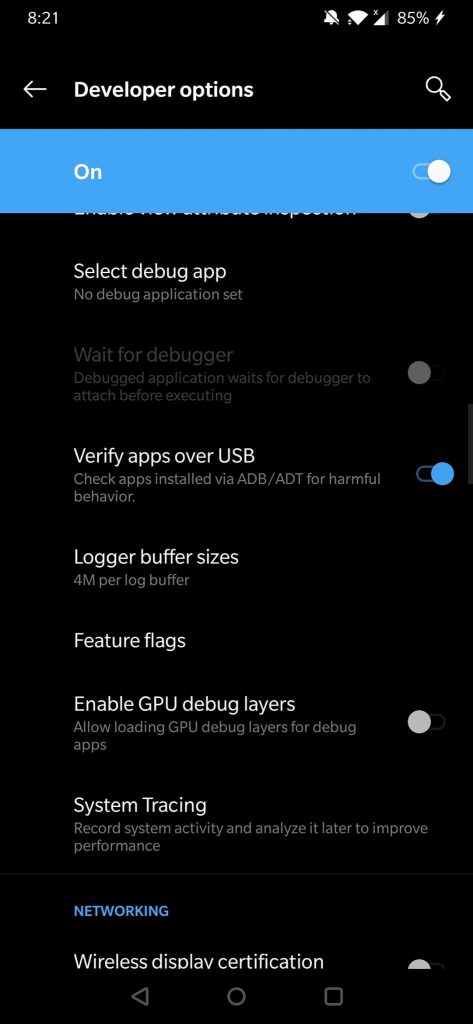A screenshot captured at 8:21 shows a mobile device's "Developer Options" settings screen. Key indicators include a battery level of 85%, excellent network service, and a muted sound setting. The screen features a heading for "Developer Options" with navigational icons such as a back arrow and a magnifying glass for search. A prominent blue "On" toggle indicates that Developer Options are enabled, while the other elements on the screen are against a black background. Specific settings highlighted in the screenshot include:

- "Select debug app" with the text "No debug application set."
- "Wait for debugger," which is disabled (grayed out).
- "Verify apps over USB" and "Check apps installed via ADB" are enabled.
- Several options such as "Logger buffer sizes," "Feature flags," and "Enable GPU debug layers" are visible, with "Enable GPU debug layers" turned off.
- "System tracing" and the category "Networking" are present.
- The "Wireless display certification" option is not enabled.

Navigation buttons are visible at the bottom of the screen.